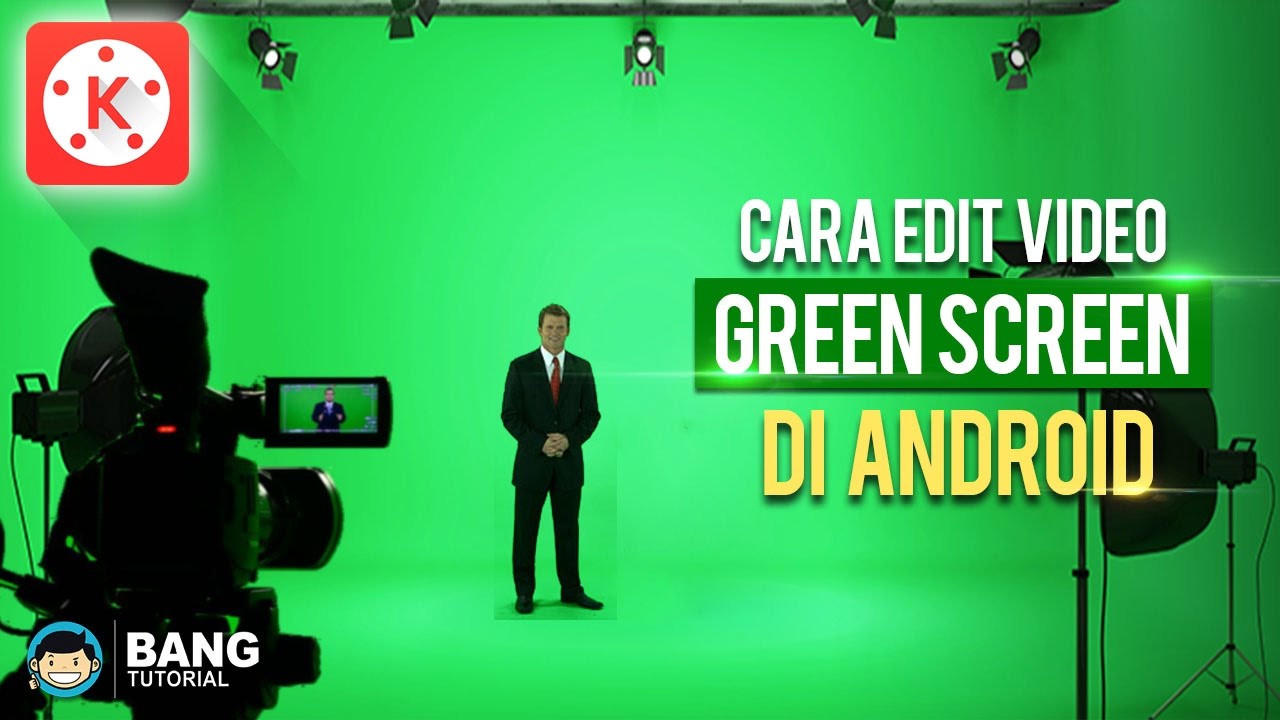A man stands slightly left of center in front of a green screen, wearing a dark suit, white shirt, and red tie. He is illuminated by several lights hanging from the ceiling and surrounded by various camera equipment, including a camera on the left that displays his image on its screen with a red recording light on. To his right, white text reads "How to Edit Green Screen Videos on Android." The top left corner features a logo consisting of a white circle with five red dots around a red letter "K," all inside a red rounded square. In the bottom left corner, white text says "Bang Tutorial" alongside an icon of a man’s cartoon face with black hair. Additionally, the caption includes "Kara edit video, green screen," in white font and "DI Android," in gold font, highlighting the tutorial's subject on editing green screen videos using Android.